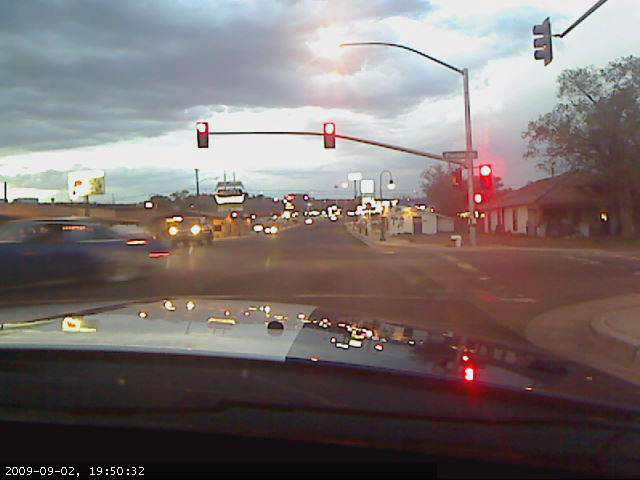From the interior of a vehicle, possibly a bus, stopped at a traffic light, we observe the dashboard, which is illuminated by numerous indicator lights and a prominent, though overexposed, red light displaying the number three. The scale and layout of the dashboard suggest it may not belong to a standard car, reinforcing the likelihood that this is inside a bus. A time stamp indicates the date as September 2, 2009, and the time as 19:50:32.

The vehicle is halted at a major four-way intersection, with the traffic light currently red. Across the intersection, a street pole extends an arm over the road, supporting two red traffic lights, with an additional red light mounted on the pole itself. Adjacent to the traffic signals is a pedestrian walk sign facing the cross street. Below the traffic lights, a green street name sign is visible, yet unreadable due to its small size and lack of focus.

The scene appears to be set during dusk, as the sky still holds some light with the sun likely about 15 degrees above the horizon. The area looks like a bustling fast food corridor, featuring illuminated signs and brightly lit buildings, contributing to the well-lit ambiance despite the approaching evening.